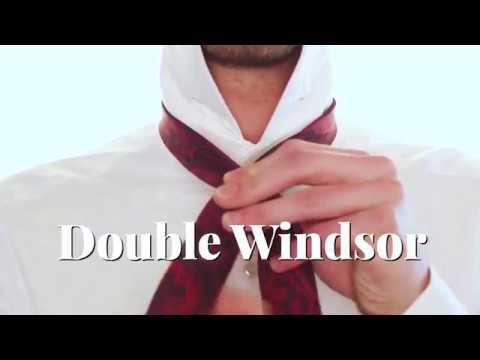This image appears to be a YouTube thumbnail for an instructional video on how to tie a Double Windsor knot. It features a white male with dark stubble on his chin, shown from the chin down to the upper chest. He is wearing a white Oxford shirt with the collar popped up to reveal a deep red tie adorned with black, potentially floral, embellishments. The person's left hand is holding the knot of the tie, suggesting he is in the process of tying it, and there is slight motion blur indicating action. The instructional nature of the video is highlighted by the text "Double Windsor," written in white with a black border, superimposed across the lower one-third of the image. The background is white, adding to the clarity and instructional focus of the thumbnail.